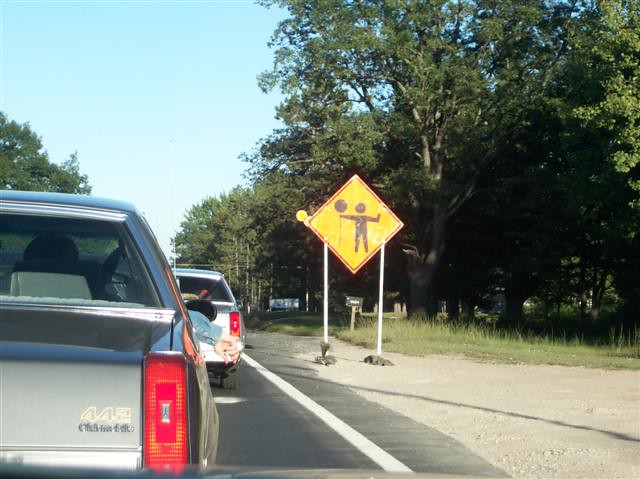This photograph captures a street scene showcasing a traffic control sign on the side of the road. The image prominently features a bright orange, diamond-shaped sign with a black border, held up by two white poles anchored with black sandbags. The sign bears an illustration of a figure with a round head and horizontally outstretched arms holding a black ball attached to a string, indicating a stop signal for motorists. In the foreground, the asphalt road is marked with a white stripe along its edge. Two older model cars are visible, stationary in front of the camera, suggesting that traffic has been halted. The overall scene, with the vintage vehicles, hints that the photograph was taken some years ago.